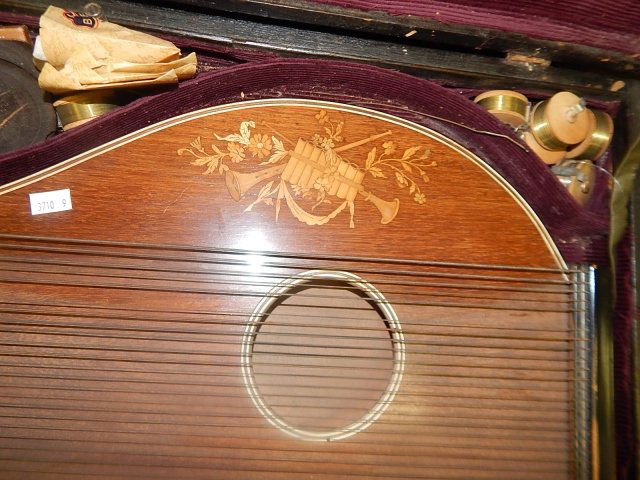This photograph captures a detailed view of a wooden musical instrument with numerous metal strings, far more than a typical guitar, suggesting it might be a mandolin or a similarly complex stringed instrument. The instrument is enclosed in a velvety maroon or burgundy case, and both the instrument and case are situated within a larger black wooden box. The instrument features an intricate design along its lighter brown surface, including illustrations of crossed trumpets, flowers, leaves, and a xylophone-like object. A doily detail is also present in the illustration. Dominating the center of the instrument, a circular soundhole is bordered in white, as is the instrument’s edge. A white sticker on the left side of the instrument, inscribed with "3710 9", hints that it might be for sale. Surrounding the case are additional elements such as light brown chair wheels with gold bands and some beige paper bags, adding to the composition's rich visual detail.